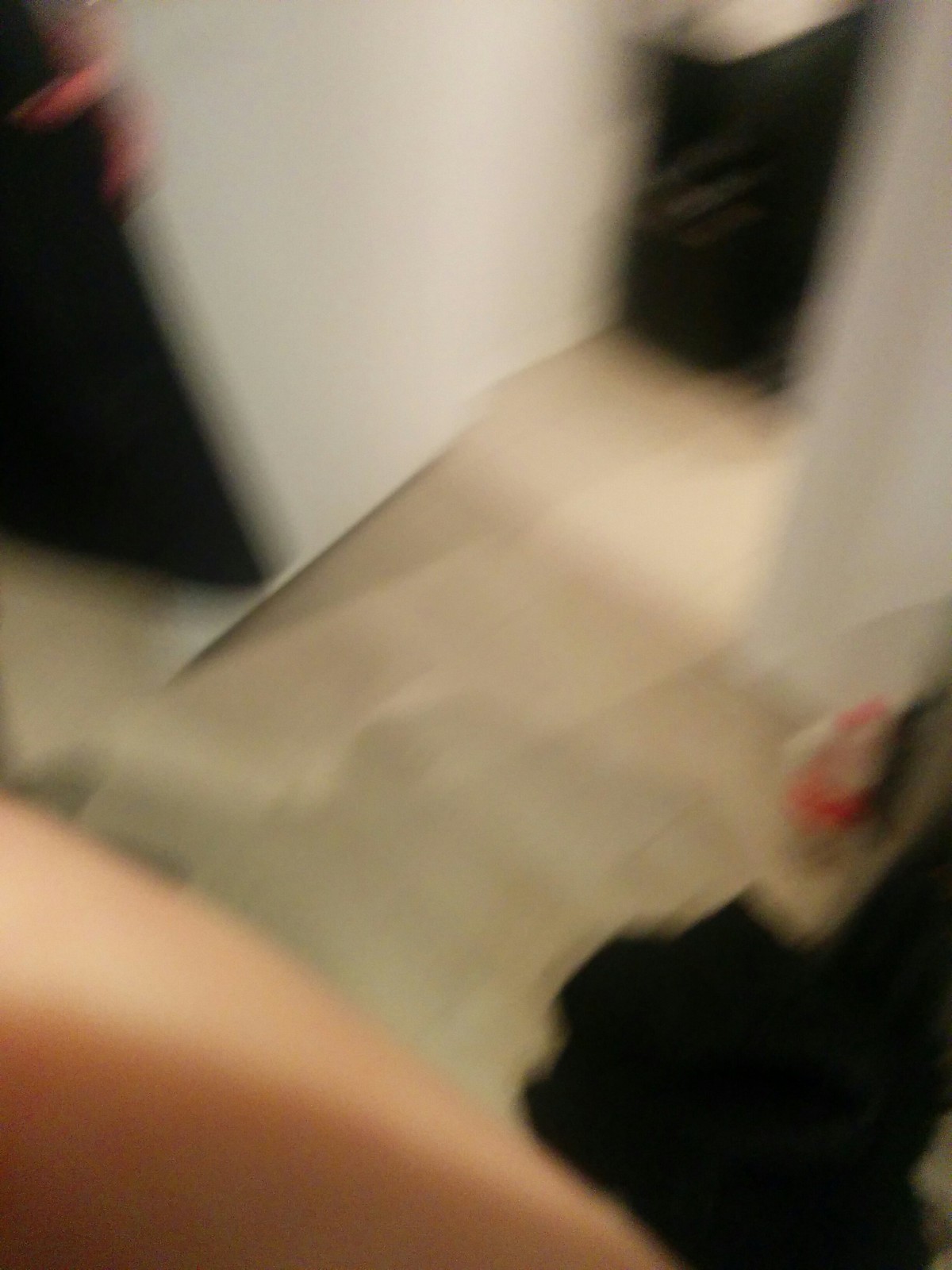The photograph is extremely blurry and depicts an indoor setting with a mix of indistinct objects and features. In the lower right-hand corner, the image shows a Caucasian arm, occupying about a third of the photo. Adjacent to the arm is a black object, possibly part of a shirt or another item. The floor appears to be a light brown color, though it's difficult to ascertain details due to the blurriness. The walls in the background seem to be white or light gray. Towards the bottom right corner, there's a faint suggestion of an empty two-liter bottle on the floor. In the mid to upper left side of the photograph, there's a rectangular black shape, potentially a doorway or a wall hang like a tapestry. Furthermore, the upper left corner has a partially visible black triangular shape with a slight red tinge on one side. The center of the image features a mix of white and light brown tones, with a prominent black streak running through the middle.